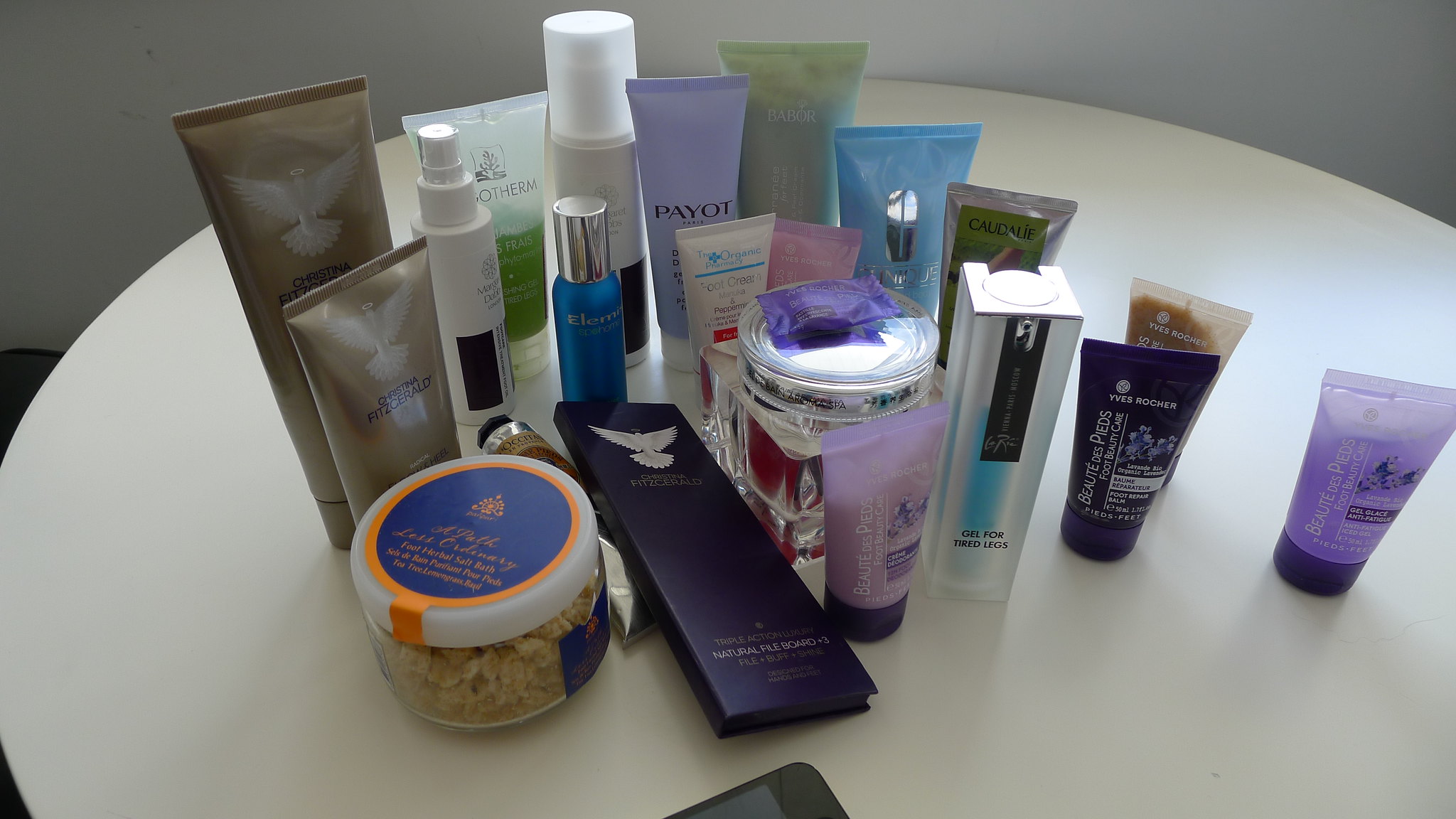In a photograph of a white, reflective table set in a well-lit room with a dark floor, a diverse array of beauty products is meticulously arranged. The products come in various colors, including purples, blues, reds, tans, browns, and whites, creating a vibrant display. Among the items is a circular container with a prominent orange-lined rim featuring blue and orange writing. It holds a chunky, tan substance and is clear in design. Another notable item is a square, navy blue product adorned with an image of a white bird. Numerous bottles, possibly lotions, are also present, varying in color from light purple with floral designs to dark blue and light brown. Particularly eye-catching is a purple bottle labeled "Payette."